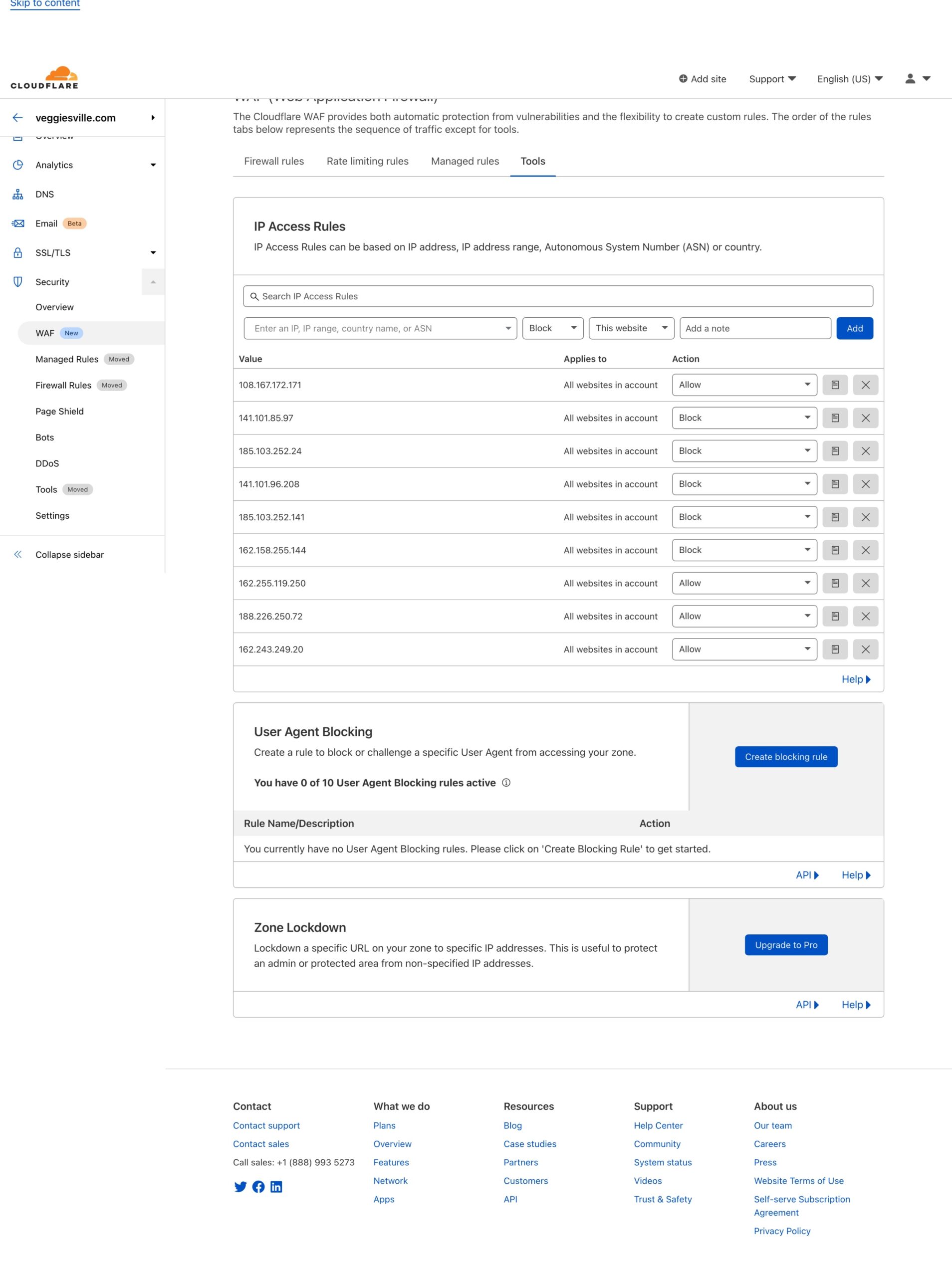The image appears to be a screenshot of a detailed computer interface related to IP access management for the website "veggievile.com," noticeable but difficult to see in the upper left due to very small text. The predominant colors in the screenshot are blue and orange, with several areas of text and button labels.

At the center of the image, there is a list titled "IP Access Rule" displaying approximately ten different rules, each accompanied by a value and action status. The action statuses are split evenly between "allow" and "block." These rules likely pertain to network security measures, determining whether specific IP addresses are permitted or restricted.

Prominently displayed in blue are actionable items: "Add," "Create Blocking Rule," and "Upgrade to Pro." These options suggest functionalities for modifying IP rules or enhancing the service.

At the top, the interface includes a header bar featuring additional navigation options such as "Add Info," "Support," and language settings denoted as "English (US)". There is also an avatar icon, presumably for user profile access.

Other noteworthy elements include mentions of "User Agent Blocking," "Zone Lockdown," and "IP Access Rules," indicative of a comprehensive security or network management tool, likely a part of a broader cybersecurity or administrative system. Additionally, there is an orange section with text that is unreadable, possibly highlighting important alerts or status indicators.